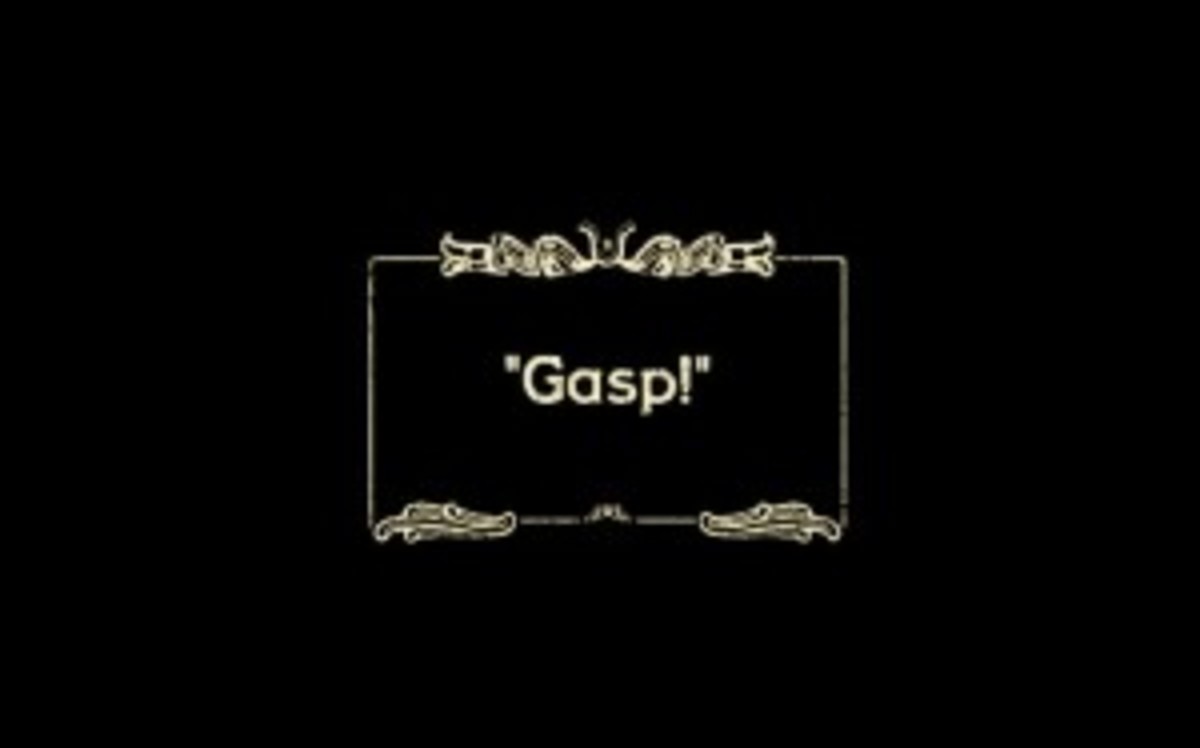The image features a rectangular box with ornate filigree decorations at the top and bottom, set against a solid black background. Inside this box, rendered in a light gold color, is the word "GASP!" in uppercase letters, enclosed within quotation marks. The text and design appear slightly blurred, reminiscent of old-time silent films that used visual cues in place of audio. This evocative, vintage style captures the essence of a bygone era of cinema, specifically highlighting the silent film era's use of intertitles to convey emotion and dialogue.